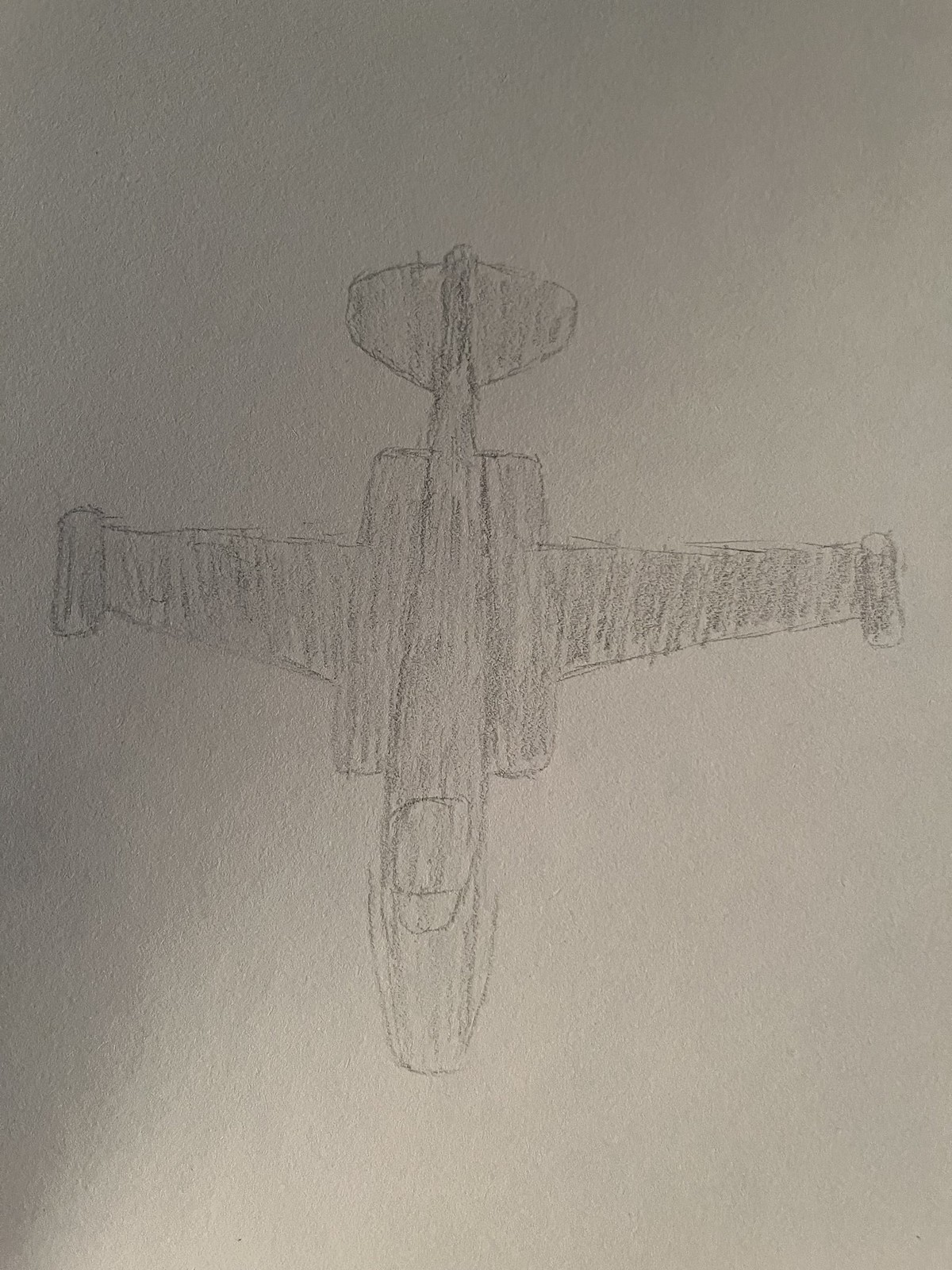A minimalist pencil sketch of a single-seater airplane graces this off-white sketch paper. The aircraft is depicted from an aerial perspective, with its nose pointed towards the bottom of the page and the tail at the top. Rendered in dark gray pencil, the drawing features basic outlines and rough shading, capturing the essence of the plane without intricate details. Despite its simplicity, the sketch conveys the fundamental form of the aircraft effectively. Notably, the artwork is unsigned, leaving the artist's identity a mystery.